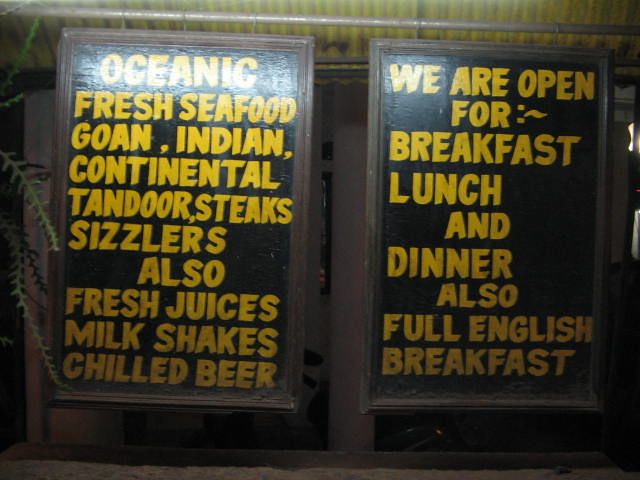This is an image featuring two rectangular signs side-by-side, each displaying a vibrant array of menu items in large, yellow text set against a black background, framed by brown borders. The signs list offerings such as oceanic fresh seafood, Goan, Indian, continental cuisines, tandoor dishes, steaks, sizzlers, fresh juices, milkshakes, chilled beer, breakfast, lunch, and dinner options, including a full English breakfast. These signs hang slightly downward from an elevated, rusty rod, which is just below the roofing structure of a restaurant or café, though the roof itself is cropped out of the image. On the left side of the photo, a few tree branches are visible, adding a touch of natural detail to the scene.